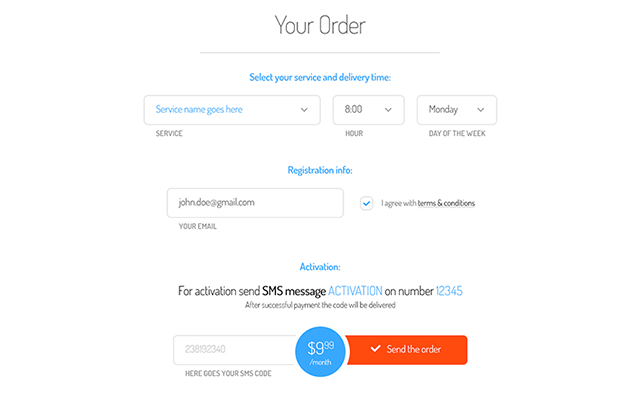This image depicts an order form from an unspecified website, featuring a blend of blue and black text. At the top, it clearly states "Order." Below, the form displays various fields pertinent to a service order. Key details include:

- **Service Delivery Time:** Options to select an hour in what appears to be a 24-hour format (as no AM/PM designation is present) and a day of the week, specifically indicated as Monday.
- **Registration Information:** An email input field is shown with the placeholder "john.doe@jiba.com," and next to it is a checkbox labeled "I agree with terms and conditions" that has a blue checkmark.
- **Activation Instructions:** There is a directive to send an SMS message for activation to the number "12345." It states that after successful payment, an activation code will be delivered.
- **SMS Code Field:** An SMS code placeholder currently shows "238192340."
- **Pricing and Order Submission:** The form indicates a cost of "$9.99 per month" and includes a "Send Order" button, suggesting the final step to complete or submit the order.

Overall, the form appears to facilitate ordering a digital service or product, possibly related to phone services, given the SMS activation requirement.